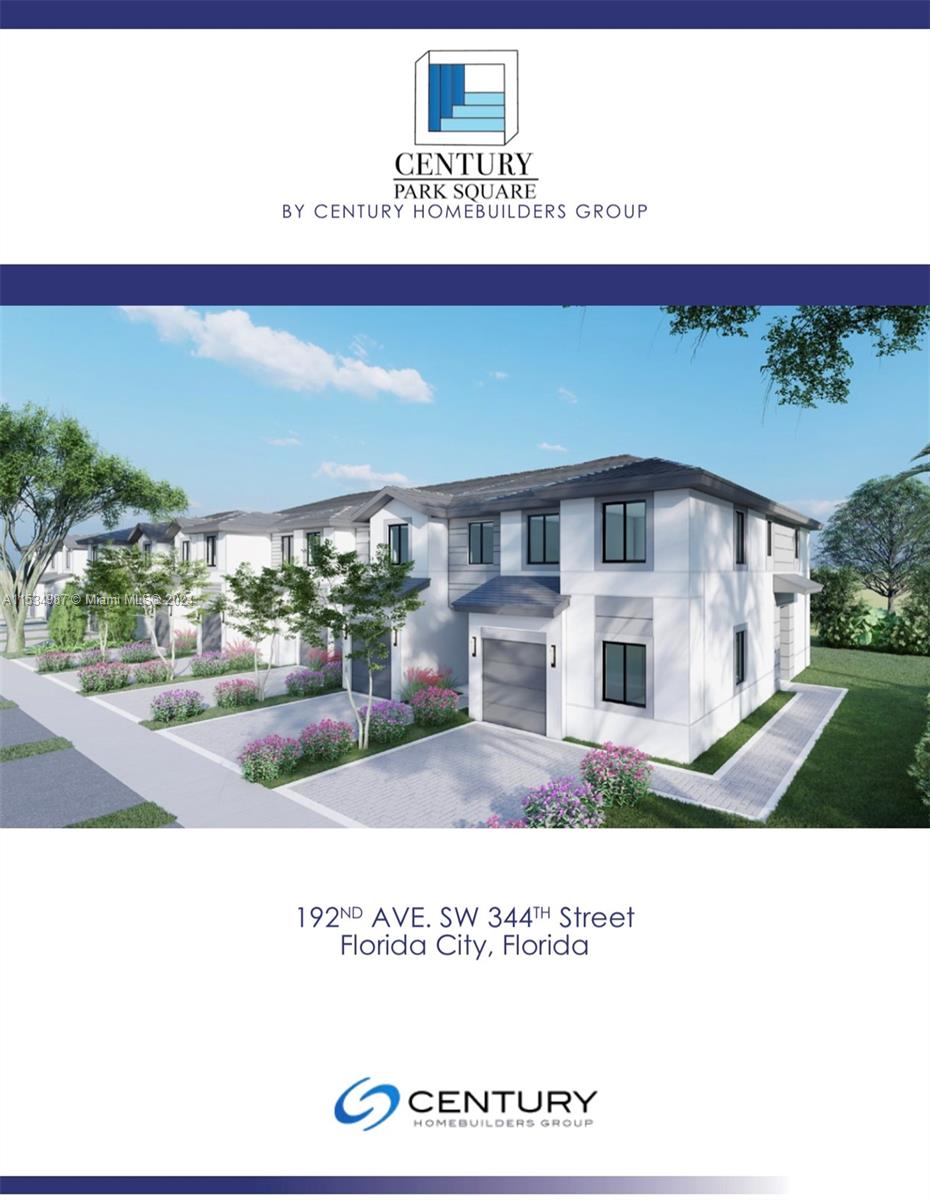The marketing magazine cover for Century Park Square by Century Home Builders Group features a prominently displayed white and dark blue graphical theme. The top of the cover showcases the company's name and logo—a white square with blue details. Central to the cover is a digitally rendered image of a townhouse-style community, with multiple connected two-story homes. Each home has a white facade, large windows, and individual garages; the driveways are separated by flower bushes and small trees. In the background, the sky is depicted as blue with scattered white clouds, enhancing the suburban feel. Below the image, the address "192nd Avenue Southwest 344th Street, Florida City, Florida" is listed, along with an additional display of the company's name and its swirling blue logo. This detailed presentation illustrates the cohesive and well-planned community of Century Park Square.